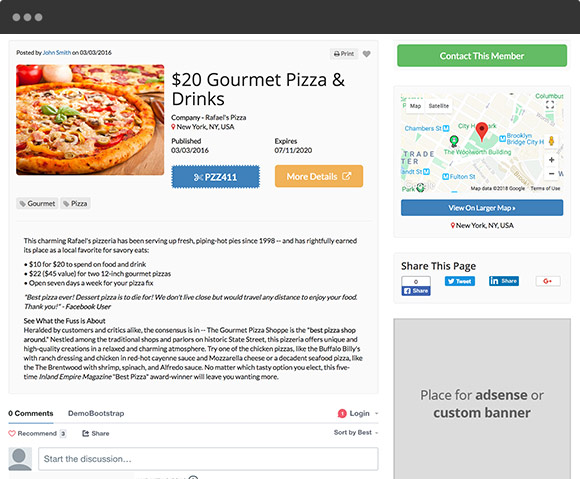### Detailed Caption for the Coupon-Style Website Image

The image showcases a coupon-style webpage meticulously designed for promotional advertising. At the top, a sleek black banner spans the width of the page, featuring three subtle gray dots situated in the upper left-hand corner, possibly indicating a menu or navigation option.

Directly below the banner, a prominent gray box holds the featured content. Within this box, there is an eye-catching image depicting two delectable pizzas arranged on a rustic table alongside an onion and a tomato. The image is accompanied by text detailing a special offer: "$20 for gourmet pizza and drinks." The offer is from Raphael's Pizza, a renowned pizzeria based in New York, New York, United States. The timestamp indicates that the offer was published on March 3, 2016, and is set to expire on July 11, 2020. The coupon code provided is "PZZ411." The tags associated with this coupon are "gourmet" and "pizza."

Additional information beneath the coupon reveals the pizzeria's reputation and offerings. Raphael's Pizzeria, established in 1998, has become a beloved local gem, known for its "Safer Eats" and various deals such as "$10 for $20 to spend on food and drink" and "$22 for $45 value for two 12-inch gourmet pizzas." The pizzeria boasts a welcoming atmosphere, open seven days a week, and is famous for its exceptional pizzas and dessert offerings. A glowing testimonial from a Facebook user praises the pizzeria's irresistible dishes, highlighting that it's worth traveling any distance for their pizza.

The page further elaborates on Raphael's acclaim, recognized by both customers and critics alike as the finest pizza shop around. Nestled among the traditional shops and parlors on the historic Straight Street, Raphael's offers a unique array of high-quality pizzas in a relaxed and charming environment. Patrons can enjoy specialty pizzas like the "Buffalo Billy," topped with ranch dressing, chicken, red hot cayenne sauce, and mozzarella cheese, or the luxurious "Brentwood," adorned with shrimp, spinach, and Alfredo sauce. Raphael's Pizzeria has earned the prestigious Inland Empire Magazine Best Pizza Award five times, ensuring every visit leaves customers craving more.

To the side, there's a section reserved for comments, encouraging user interaction. The bottom-right corner of the page is designated for AdSense or a custom banner. Additionally, a small map in the upper-right corner pinpoints Raphael's Pizza location, providing easy directions for potential customers.